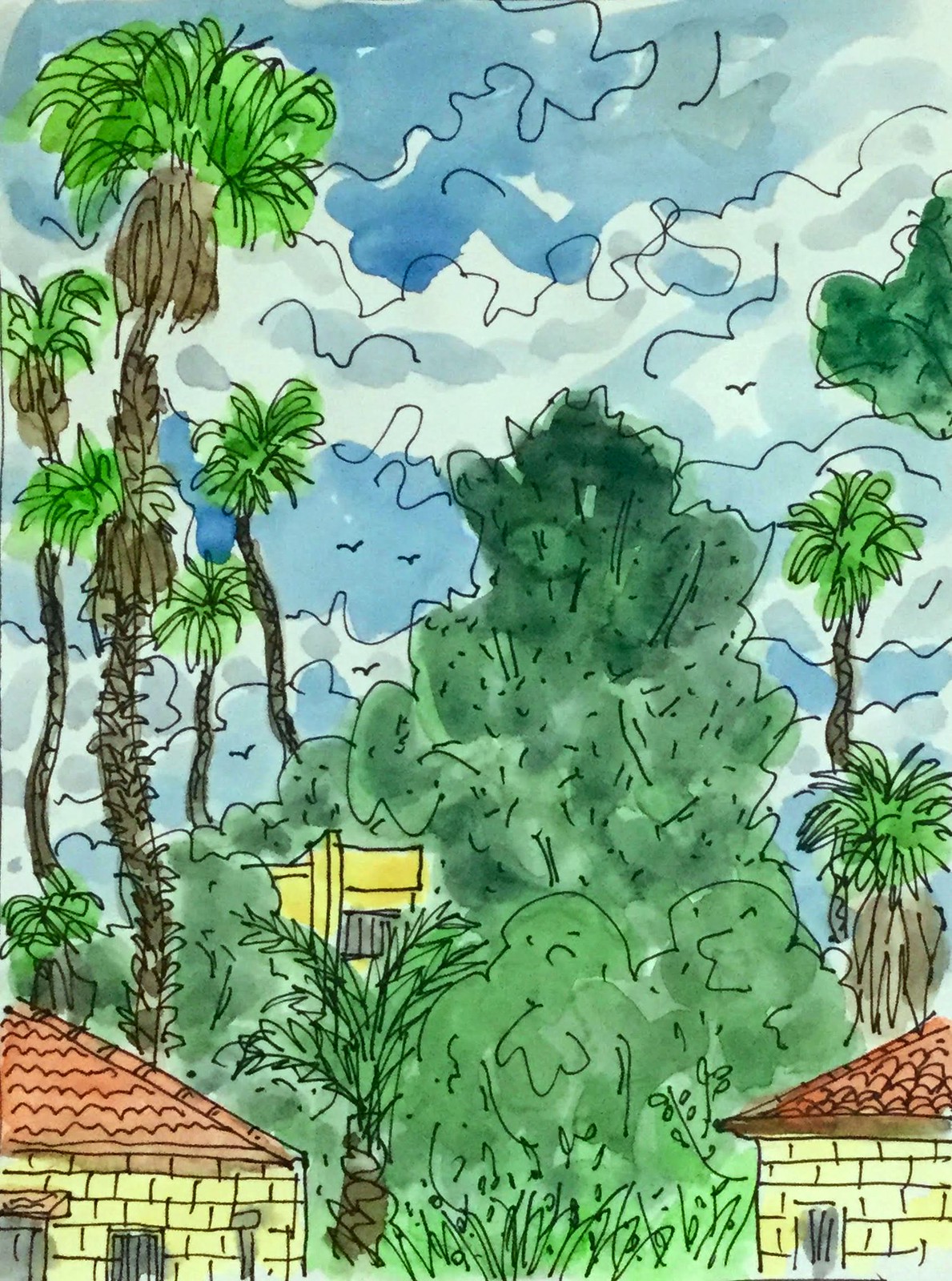A whimsical and highly stylized light watercolor pencil drawing features a charming scene. On the left, a quaint yellow brick house is partially visible, adorned with a reddish roof. The doorway, intriguingly incomplete, hints at the entrance. Mirroring this on the right side is a similar building, its detailed tiled reddish roof and open grayish door inviting the viewer's curiosity. The overall ambiance exudes a jungle-like feel, with overgrown grass dominating the foreground.

Tall, curvy, and stylized palm trees with brown trunks and dark green, fluffy leaves stretch upwards, adding to the scene's tropical atmosphere. The center of the artwork showcases lush greenery, softly outlined and rendered in transparent watercolor hues. Above, a vibrant blue sky dotted with detailed clouds completes the composition. The entire drawing has a delightful, swirly, and sketch-like quality, making it a visually captivating piece.